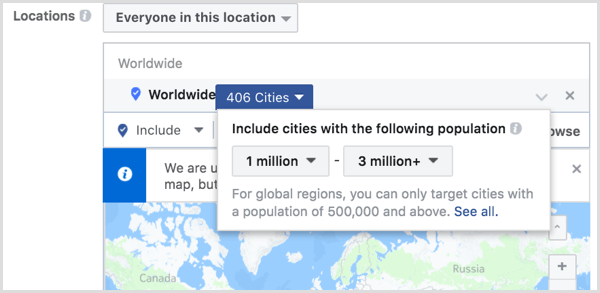The left-hand side of the image displays locations in black text on a white background. Adjacent to each location is an informational icon, represented by a white eye within a gray circle. Below this, there's a selection box labeled “everyone in this location” with a drop-down menu beside it that currently displays “worldwide.”

In the foreground, there is a pop-up covering parts of the window behind it. The background window has a checkbox feature marked with a pin icon and the text “include," accompanied by a drop-down menu. Next to this, there is another informational icon enclosed in a blue square; the circle around the "i" is white and the "i" itself is blue. The partially obscured text on this information icon reads "we are unable to..." but the rest is blocked by the pop-up. There is also a close ("X") button to dismiss the pop-up.

Beneath these elements, there is a world map prominently displaying Canada and Russia. A plus sign icon is present, allowing users to zoom in on the map. Additionally, a small square with an upward arrow suggests an export or upload function. 

Within the pop-up, the text “406 cities” is displayed on a dark blue background with white text and a white drop-down arrow. It reads “Include cities with the following population” within a white box. Further down, there are two drop-down boxes: the first reads "1 million" and the second "3 million plus," separated by a dash. The text beneath these boxes states, "For global regions, you can only target cities with a population of 500,000 and above." Finally, there is a link reading “see all” for more detailed options.